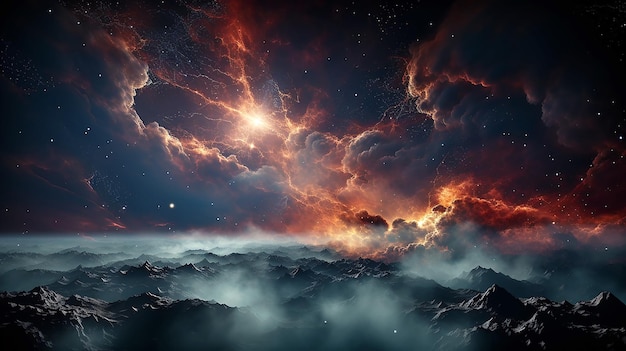This captivating image, likely AI-generated, presents a fantastical night scene reminiscent of a primordial or otherworldly landscape. At the base of the rectangular photograph, rugged, dark gray mountains with sharp peaks rise against a backdrop of swirling gray fog and dense clouds. These mountains are steeped in an eerie mist that seeps through the valleys, creating a haunting ambiance. Above this dramatic terrain, the night sky unfolds, dotted with countless stars that twinkle amidst dynamic cloud formations. The clouds are predominantly gray and blue, interspersed with vibrant streaks of pink, orange, and yellow, giving the impression of turbulent weather. Strikingly vivid lightning-like crackles or bright energy streaks traverse the sky, adding an element of dramatic intensity. The central point of the image features a bright light source—likely a star or perhaps a distant sun—illuminating the scene with a subtle yet mesmerizing glow. The image exudes a moody, sci-fi aesthetic, with the brightness fading into darker tones towards the edges, enhancing the enigmatic and surreal atmosphere of this otherworldly vista.